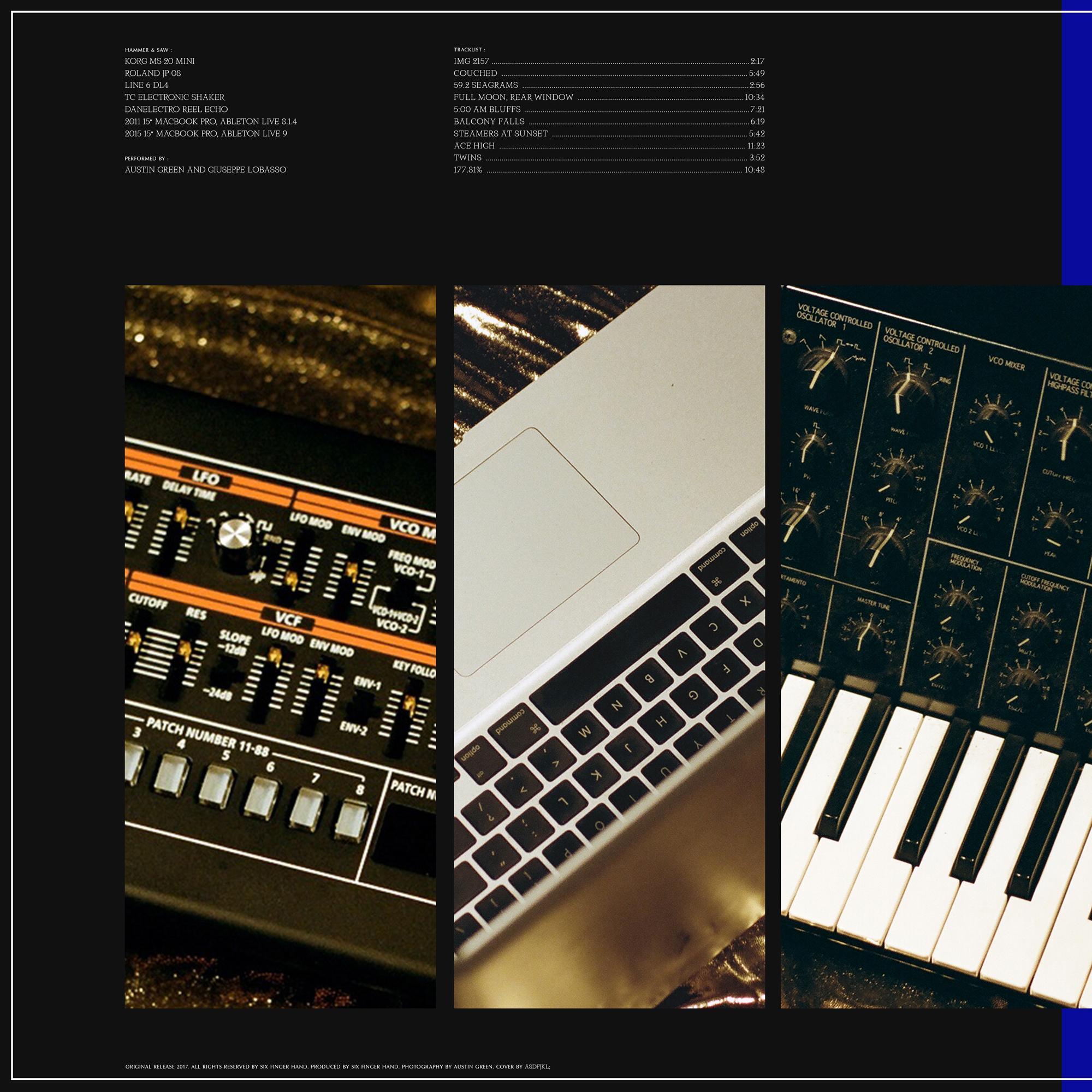Vertical image with a solid black background, featuring thin white borders along the top, left, and right edges. A thicker blue line extends from the top right corner and another blue section appears at the bottom right. 

At the top, white text lists various musical equipment and software, including: "KORG MS-20 Mini, Roland JP-06, Line 60L4, TC Electronic Shaker, Dan Electro Reel Echo, 2011 15-inch MacBook Pro, Live 1.4, Live 9." The performers, "Austin Green and Giuseppe Lobasso," are also mentioned. Additional information on track listings and song durations is provided.

The lower part of the image showcases three close-up photos: buttons of a sound device, an upside-down laptop keyboard, and a piano keyboard.